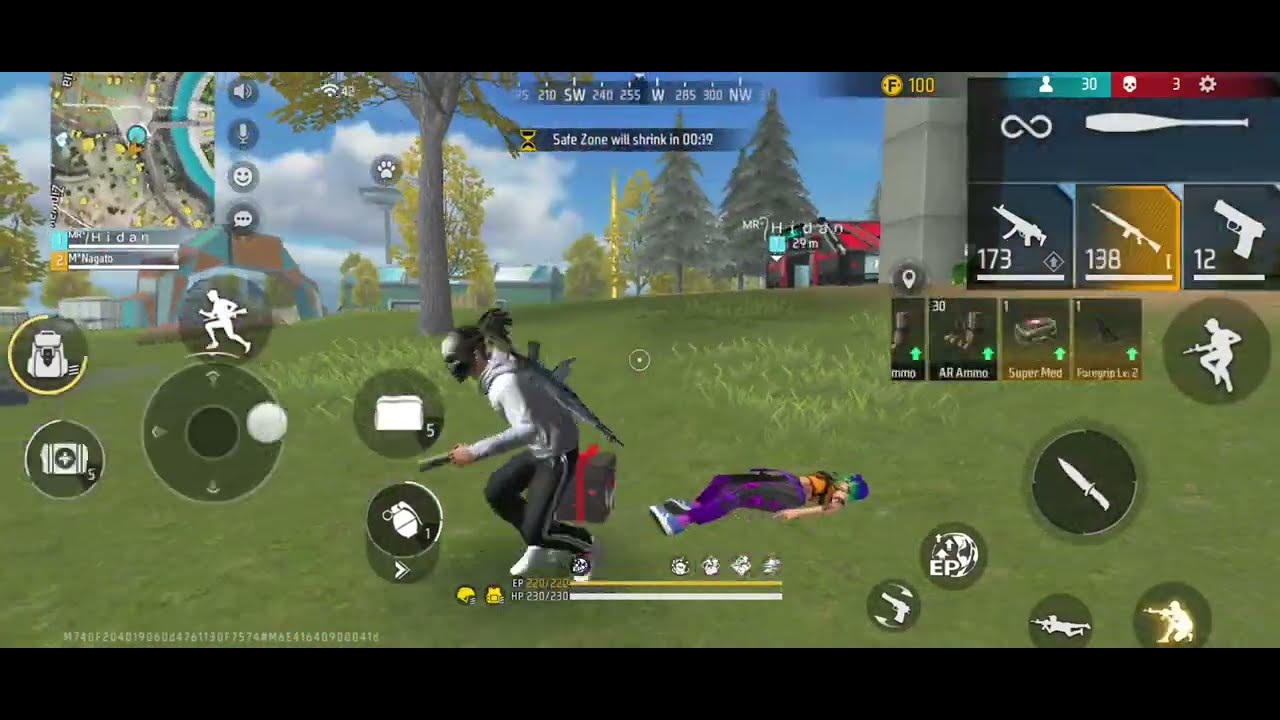This image is a detailed screenshot of a video game, potentially akin to Fortnite or a similar battle royale genre, due to the presence of a shrinking safe zone indicator. The setting is a forest scene, with visible trees and possibly a park or building in the background. The game's interface is highly detailed and busy, featuring multiple HUD elements. In the upper left corner, there's a map, while the upper right shows the player's inventory, including a bat, guns, ammo, and health stats, as well as the number of kills. The central upper section displays a compass with directions like Southwest, West, and Northwest. At the bottom left, control icons are visible, such as up, down, left, right. The main foreground character is crouching and wearing purple pants, with distinctive blue and green hair, and a face mask. This character is holding an item, with a gun slung on their back and a hand grenade visible. Behind the main character is a downed player, suggesting a recent skirmish. There's also a box or present nearby, adding to the scene's details.